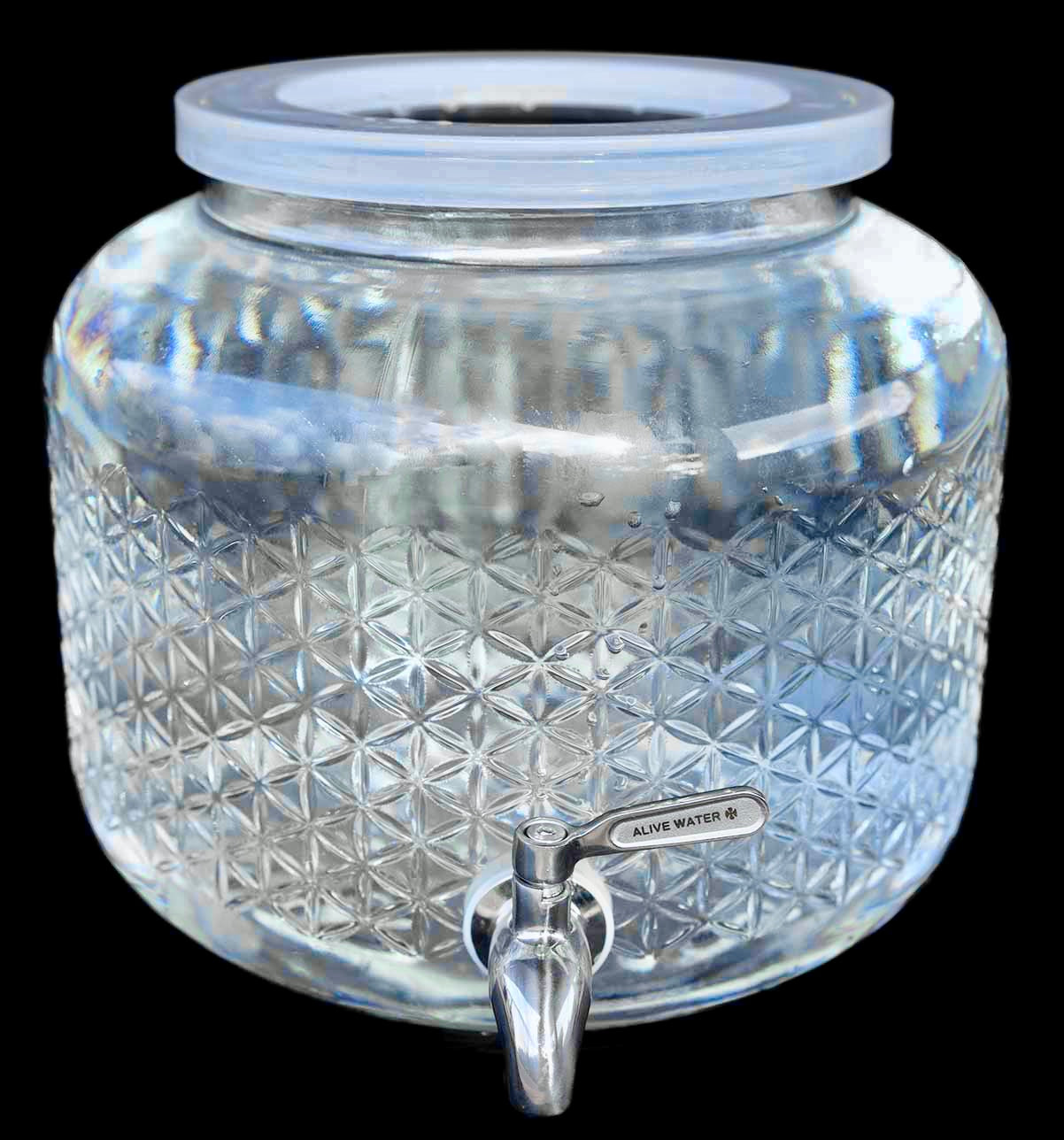This high-resolution, professionally-photographed image showcases a transparent water canister made of either glass or a glass-like material, set against a completely black background. The canister features a distinctive, almost cylindrical shape with diamond-patterned engravings along its sides, narrowing at the top. Its design includes a round, open lid for easy filling without the need for removal. A prominent, stainless steel spigot with a white handle is located at the front center of the canister. The handle is clearly labeled with "Alive Water" in black font. Although the canister appears empty, a few water droplets are visible on its interior. The sleek, modern aesthetic and meticulous detail, alongside the black background, suggest the photo was taken in a studio environment for a sophisticated and clean look.